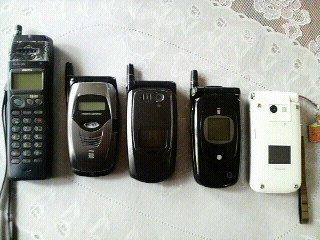The photograph is a color image of five old-school mobile phones from the early 2000s, meticulously arranged side-by-side in a row. The background features a white, almost lacy tablecloth, with a small part in the upper right corner appearing slightly transparent over a beige cloth below, while the rest seems to be white underneath. 

On the far left is the longest and tallest phone, looking particularly ancient with a green screen, a visible keyboard, and a cord coming out of the bottom; it even sports a small antenna. The second phone is silver, slightly rounder, and resembles a clamshell design, with a small green screen and a tiny antenna, possibly indicating that it might also be a flip phone. The third phone is mostly black without visible buttons, suggesting it could be a flip phone, but no screen is apparent. The fourth phone, black with a small antenna, features a larger square screen with dots above and below it, and is also likely a flip phone. The final phone on the far right is white, potentially another clamshell model, with a cord extending from its right side and possibly an orange element on the edge of the photo, and it appears to have a small square which might be a screen or other feature. 

Each phone exhibits distinct design characteristics, capturing the evolution of mobile phone design during that era.